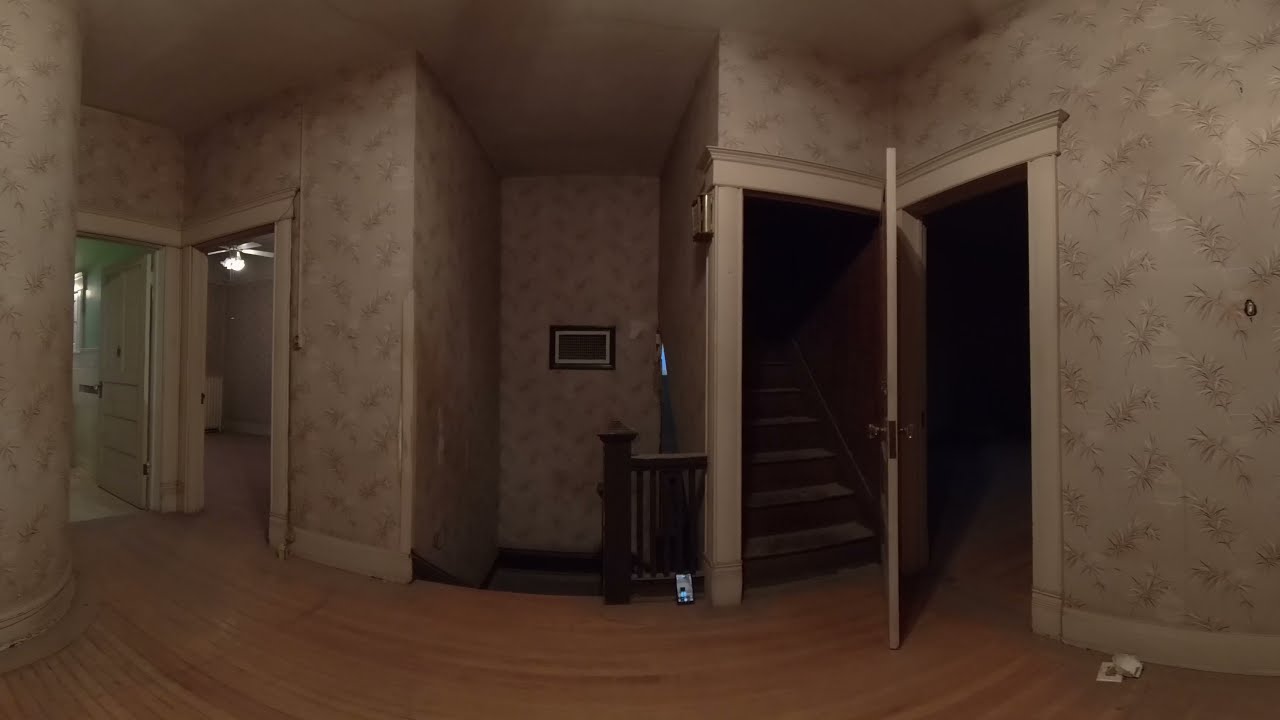This photograph captures the interior of an old-fashioned home with a distinctly vintage charm. Dominating the scene is a central post and a deep mahogany staircase leading downwards, framed by two additional staircases on either side. The wooden floors extend throughout, adding to the home's aged elegance. On the left side, two rooms with open doors reveal lit interiors, including a bathroom and a bedroom with a ceiling fan. The wallpaper, a dull cream color adorned with repetitive floral patterns and spiky leaves, lends a nostalgic feel to the setting. To the right, there's a darker room with an open door, and a staircase ascending off to the side. A framed picture hangs on the wall near the downward stairs, contributing to the quaint, slightly dim atmosphere of the house.